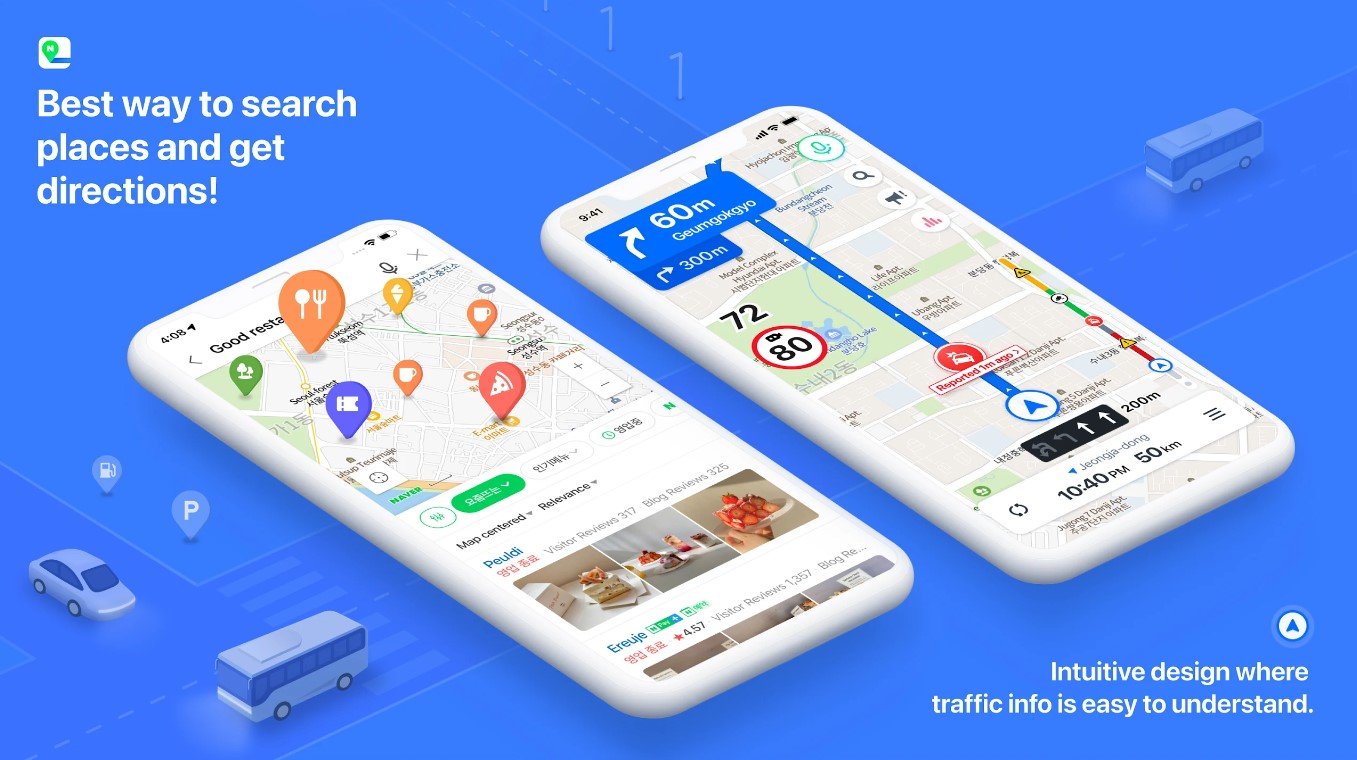The image is an advertisement featuring a vibrant blue background. In the top left corner, there's a distinctive icon: a white box with rounded edges containing a minimalistic green symbol, reminiscent of a location pin. Below this icon, bold white text proclaims, "Best way to search places and get directions!", emphasizing its promise with an exclamation point. 

Dominating the central part of the image are two white smartphones, displayed at a slight angle, showcasing various app interfaces. The phone on the left partially reveals the word "restaurants," accompanied by an orange location icon featuring a spoon and fork, symbolizing dining options. Additionally, the screen displays various other icons: a slice of pizza, two coffee cups, and a tree, suggesting categories like pizza places, cafes, and parks.

The phone on the right focuses on navigational features. It prominently displays "16m" in a blue rectangle with an arrow, indicating distance, while "80 degrees" is encased in a circle with a red border, likely indicating temperature. This screen also shows a GPS starting point with a route outline, marked by a timing of "10:40 p.m." and a distance of "50 kilometers." 

At the bottom right of the advertisement, additional text reads, "Intuitive design where traffic info is easy to understand," underscoring the user-friendly nature of the app being promoted.